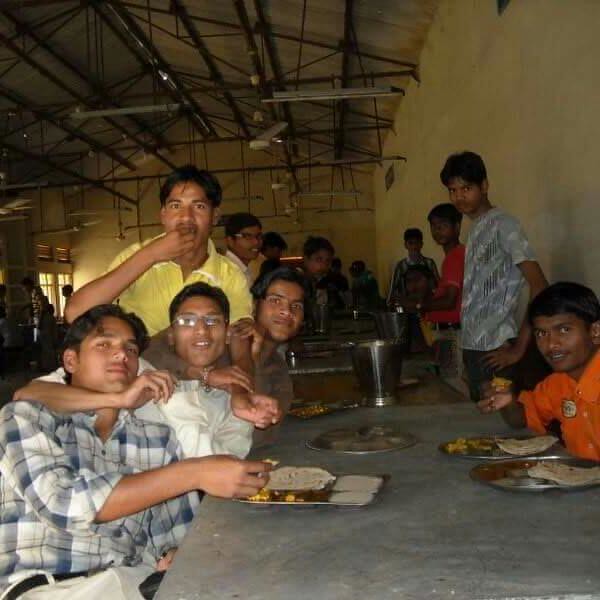The photograph captures a lively scene of young men, predominantly Hispanic or Central American, eating in a large hall that resembles a community center or warehouse. The hall has yellow walls, high ceilings with fluorescent lights, and black scaffolding near the ceiling. In the foreground, a group of four men is seated at a gray table adorned with sections of gray tablecloth. They are eating from small metal trays that each contain flatbread and other unidentifiable foods. A silver pitcher of water or another beverage is positioned on the table. 

The men, who have medium to medium-dark complexions, dark hair, and dark eyes, are dressed in a variety of Western-style clothing, including polo shirts, collared shirts, khakis, and t-shirts. They appear to be enjoying themselves, posing and laughing for the camera. In the background, many more people are visible, though their features are less discernible. Some seem to be getting food from another table, while others are sitting or standing at tables that also have silver trays and large silver buckets. Light streams in from small windows on the far back left of the hall, adding a touch of natural light to the otherwise dim room.